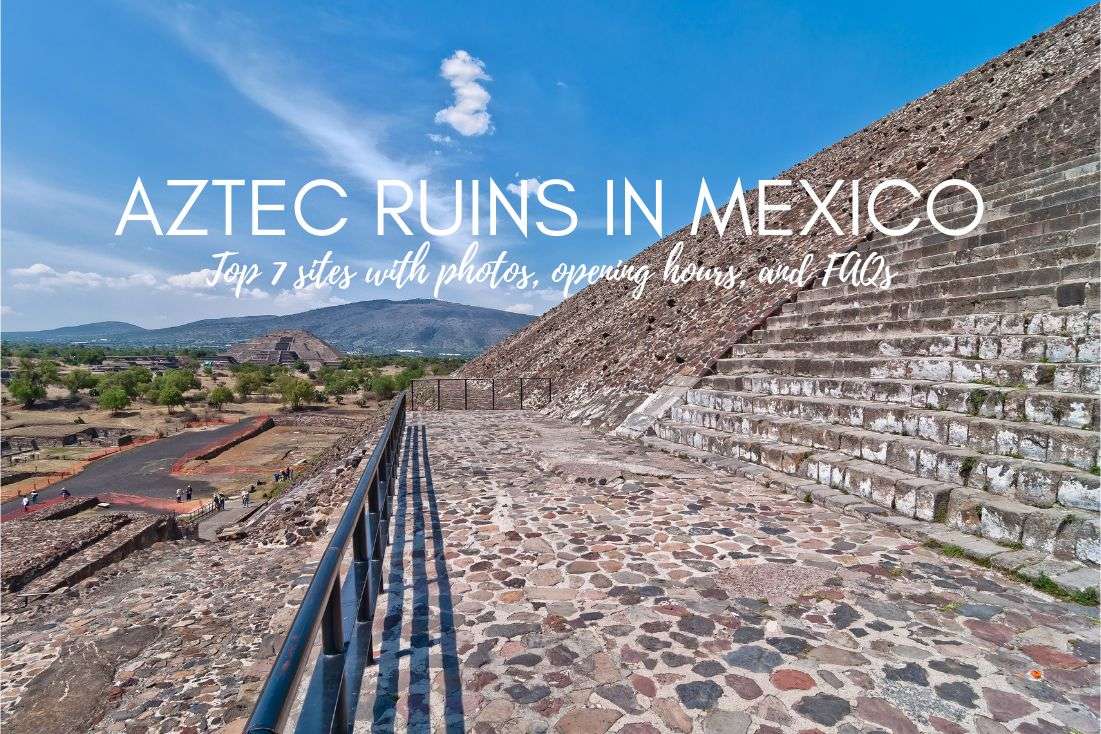The image depicts an expansive scene of Aztec ruins in Mexico, prominently featuring a stone platform that extends across the foreground. To the right, stone steps ascend a grand Aztec temple, or ziggurat, made from stones varying in color from white to reddish-brown. The platform itself is paved with cobblestones in hues of gray, red, maroon, pink, and off-white. A black metal railing lines the left side, beyond which there is an additional level down to a stone plaza. In the distance on the left, another grand stone temple is visible, set against a backdrop of towering mountains. The sky above is a clear blue, dotted with a few high-altitude clouds, especially visible on the left. Scattered visitors can be seen, particularly on the left side, appearing as small figures against the grandeur of the architecture. Overlaid on the image is white text, “Aztec Ruins in Mexico,” followed by a cursive subtitle, “Top seven sites with photos, opening hours, and FAQs,” highlighting the image’s use as an advertisement.